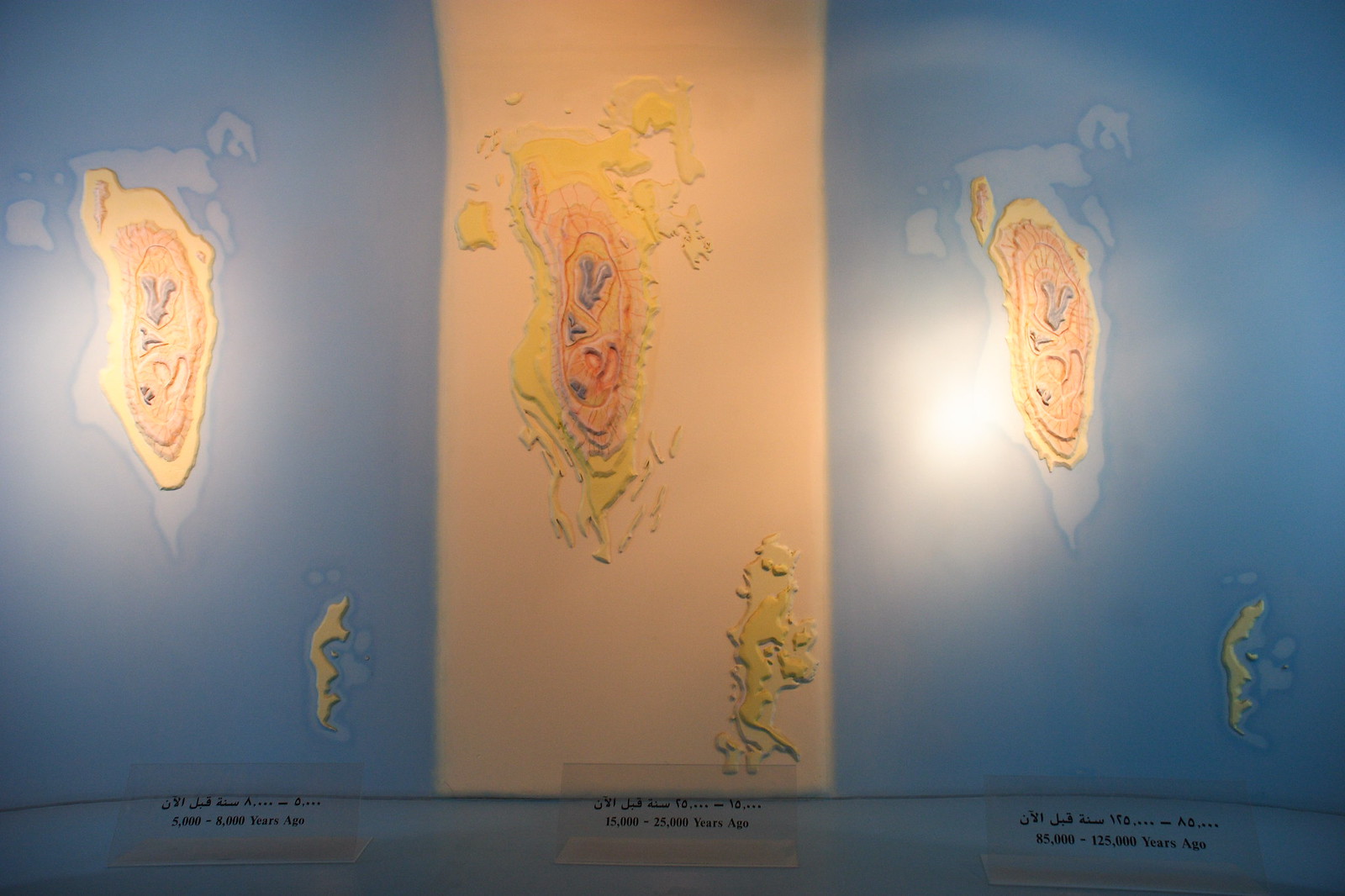The photograph depicts a detailed, illustrative display inside a museum, showcasing a brightly painted wall divided into three vertical sections. The overall color scheme features soft pastels with a central peach-colored vertical strip flanked by light blue sections on either side, which transition into oceanic themes. The wall is adorned with elliptical, landmass-like shapes rendered in a spectrum of colors, including orange, gold, purple, red, and yellow, representing different elevation levels.

In the middle section, a significant landmass stretches vertically, enveloped in soft orange hues, symbolizing varied elevations with colors transitioning from purple at higher elevations to yellow closer to the ground. The left and right sections each feature two smaller, swirly, island-like illustrations in blue tones, enhancing the oceanic theme. Among the imagery are two symbols located on the top left and bottom right of the central section.

At the base of each section are three clear plexiglass plaques. The text on these plaques is written in a foreign language and includes timeline references ranging from 5,000 to 125,000 years ago. These timelines suggest the display captures a historical representation of geographic formations over extended periods, emphasizing the museum's focus on historical geological changes. The photograph, in landscape orientation, captures the artistic representational realism of the display, blending detailed artistry and informative content.